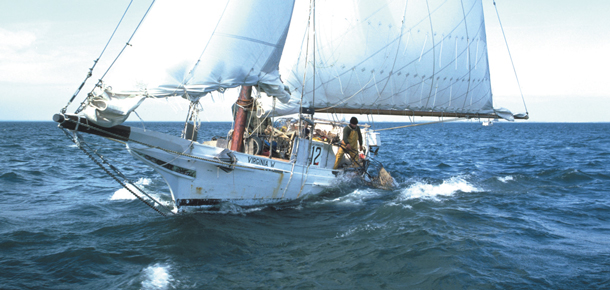In this vibrant photograph, a small white sailboat named "Virginia" glides across the shimmering blue ocean, leaning slightly to its left. The boat's bow lifts higher than the stern, with two impressive white sails catching the sunlight, particularly illuminating the sail on the left. A person is depicted near the back of the boat, reaching into the water, seemingly pulling up a substantial fish. The ocean is adorned with white caps, and the clear sky above features light blue hues and scattered white clouds. The boat also bears a number on its side, including the digit "2," in black text, visible beneath the dazzling brightness of the day.